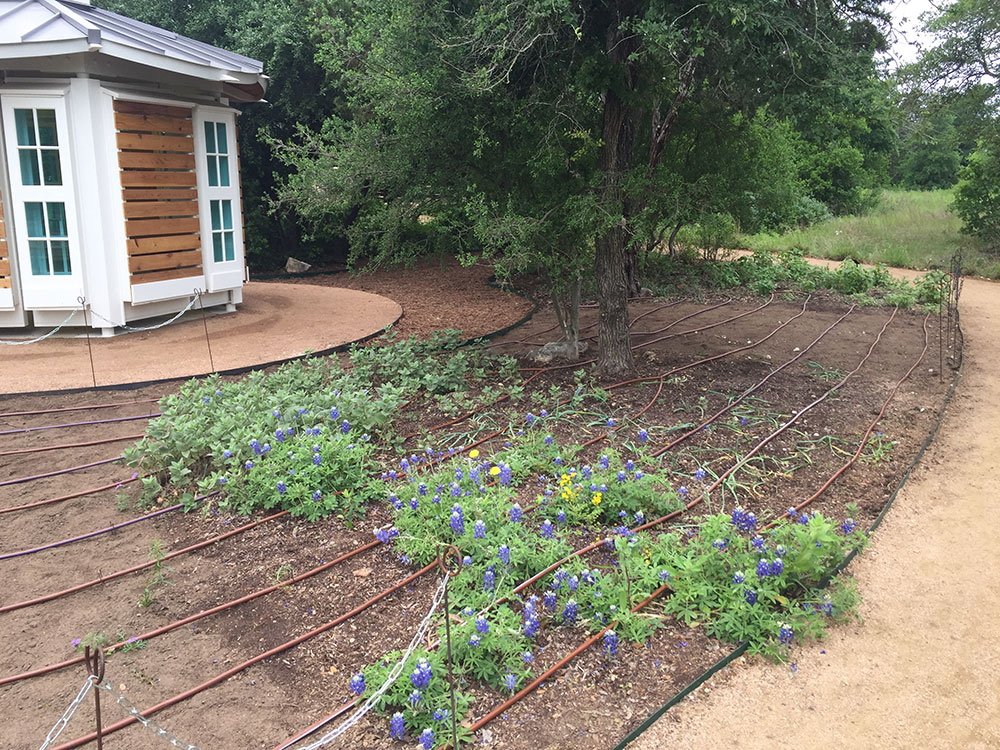The photo captures a picturesque garden scene situated in a forest-like setting, potentially within a national preserve or park, as suggested by the numerous surrounding trees and a fence enclosing the area. Dominating the upper left of the image is a small, white and gray wooden garden shed or cottage with a brown door and a gray roof. It features four white-trimmed windows and measures approximately 100 square feet. 

In the foreground, an array of vibrant purple flowers, interspersed with yellow dandelions and other assorted blooms, flourish. These flowers are laid out in rows, forming a circular pattern, with irrigation lines snaking through them to ensure they are well-watered. There is also a mix of green shrubs and large green trees surrounding the garden area, adding to the lush, natural vibe. A sandy trail weaves around the garden, which contains patches of freshly tilled soil, suggesting recent gardening activities. Overall, it is a delightful blend of wild and cultivated flora within a serene, wooded environment.